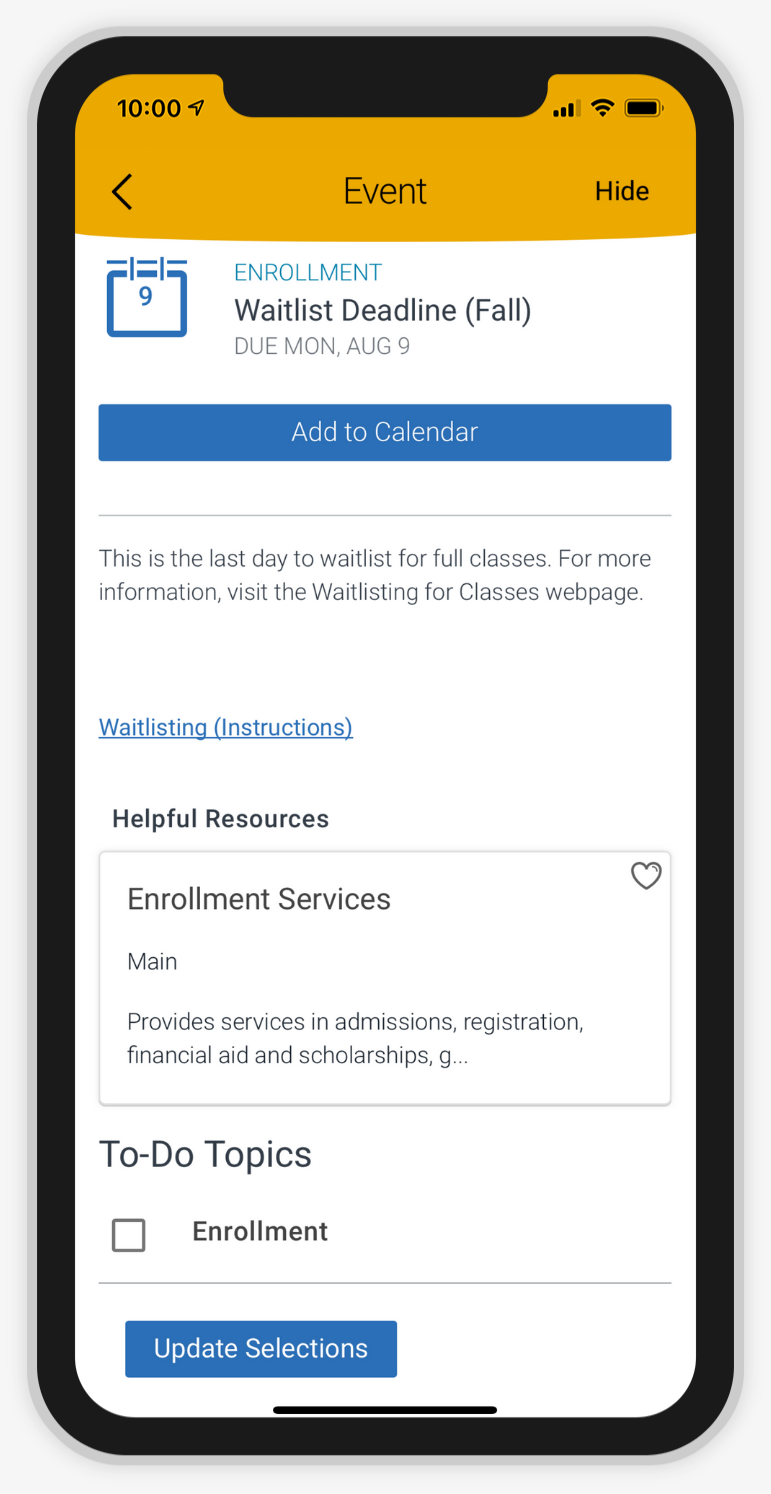The color image appears to be a photograph of an iPhone displaying a website formatted for mobile viewing. The iPhone is identifiable by a noticeable black notch at the top and a black curved rim along the edges of the phone. The screen is predominantly occupied by a yellow-orange banner featuring black text. At the top left, the banner shows the time as 10:00, a back arrow event indicator in the center, and a "hide" option on the right. Above the banner, various mobile icons are visible, including a Wi-Fi signal icon and a fully-charged battery icon.

Directly below the banner, the background shifts to white with mostly black text. The top section highlights key details such as "Enrollment, waitlist, deadline of fall," and a due date of August 9th. To the right, there's a rectangular icon with a line resembling something hanging from a pole. Below these details, a prominent blue button labeled "Add to Calendar" is followed by a thin horizontal grey line. 

The subsequent text alerts readers that "This is the last day to waitlist for full classes" and directs them to visit the "waitlisting for classes webpage" for more information. Further on, there are blue, underlined "waitlisting instructions." Continuing down, another section titled "Helpful Resources" is displayed, featuring a rectangle marked "Enrollment Services" with a heart icon in the upper right-hand corner. This section includes a brief description stating "Main, Provide services in admissions, registration, financial aid and scholarship. G..."

Towards the bottom, there are two to-do topics, one of which is an unticked square box labeled "Enrollment." Finally, at the very bottom of the webpage, a blue rectangular button with the text "Update Selections" in white is visible.